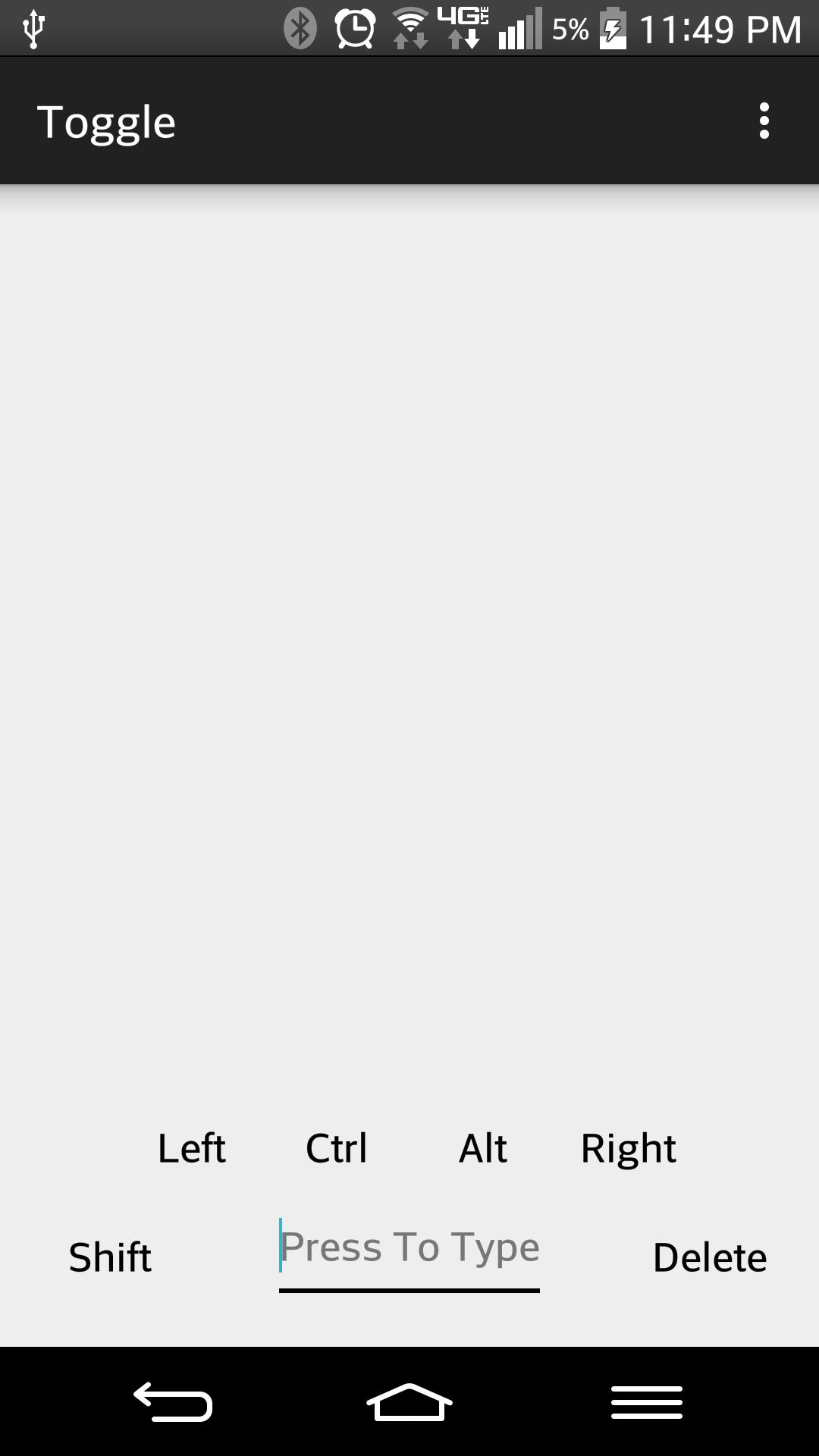The screenshot from a cell phone shows a detailed interface with various elements. In the upper right corner, the time is displayed as 11:49 p.m. Adjacent to it, on the right side of a black bar, there are three vertical dots for additional settings or options. To the left of this bar is the word "Toggle" in white text.

Below the black bar, the main screen area is predominantly gray and blank until the bottom part, which features two rows of text. The first row contains the words "Left Ctrl," "Alt," and "Right" in black text. The second row reads "Shift," "Press to type," and "Delete," with "Press to type" in gray, underlined text. A blue line is present to the left side of the "P" in "Press," indicating an editable text field.

At the very bottom of the image, there is another black bar housing three distinct symbols: a backward C-shaped arrow pointing to the left on the left side, a house icon in the center, and three horizontal lines on the right side, representing different navigation or action options.